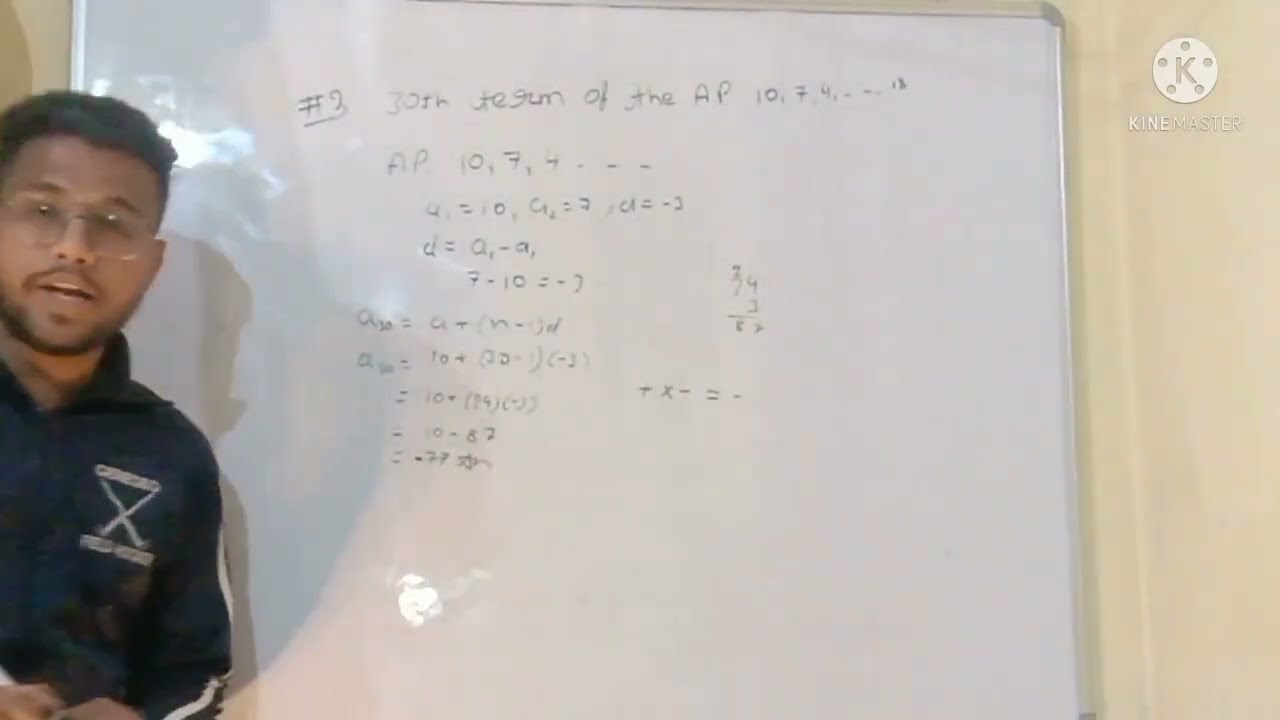A man of Middle Eastern descent, possibly Indian or black, stands in front of a whiteboard, delivering what appears to be a math lesson for an online video or livestream. He has short hair, wears glasses, and sports a goatee. Dressed in a black long-sleeve shirt with a white stripe down his arm and an 'X' on his chest, he is positioned on the left side of the image, engaging the camera as he explains the content. The whiteboard behind him, mounted on a tan wall with a silver outline, features an unreadable equation written in black marker. Prominently displayed at the top of the whiteboard is "KineMaster," along with a K inside a circle. Although the specific details of the math problem are unclear due to his handwriting, the visible text includes elements such as "number 3," numerous arithmetic sequences, and various algebraic expressions and operations. The scene suggests an educational setting, likely part of a streaming or recorded math tutorial.